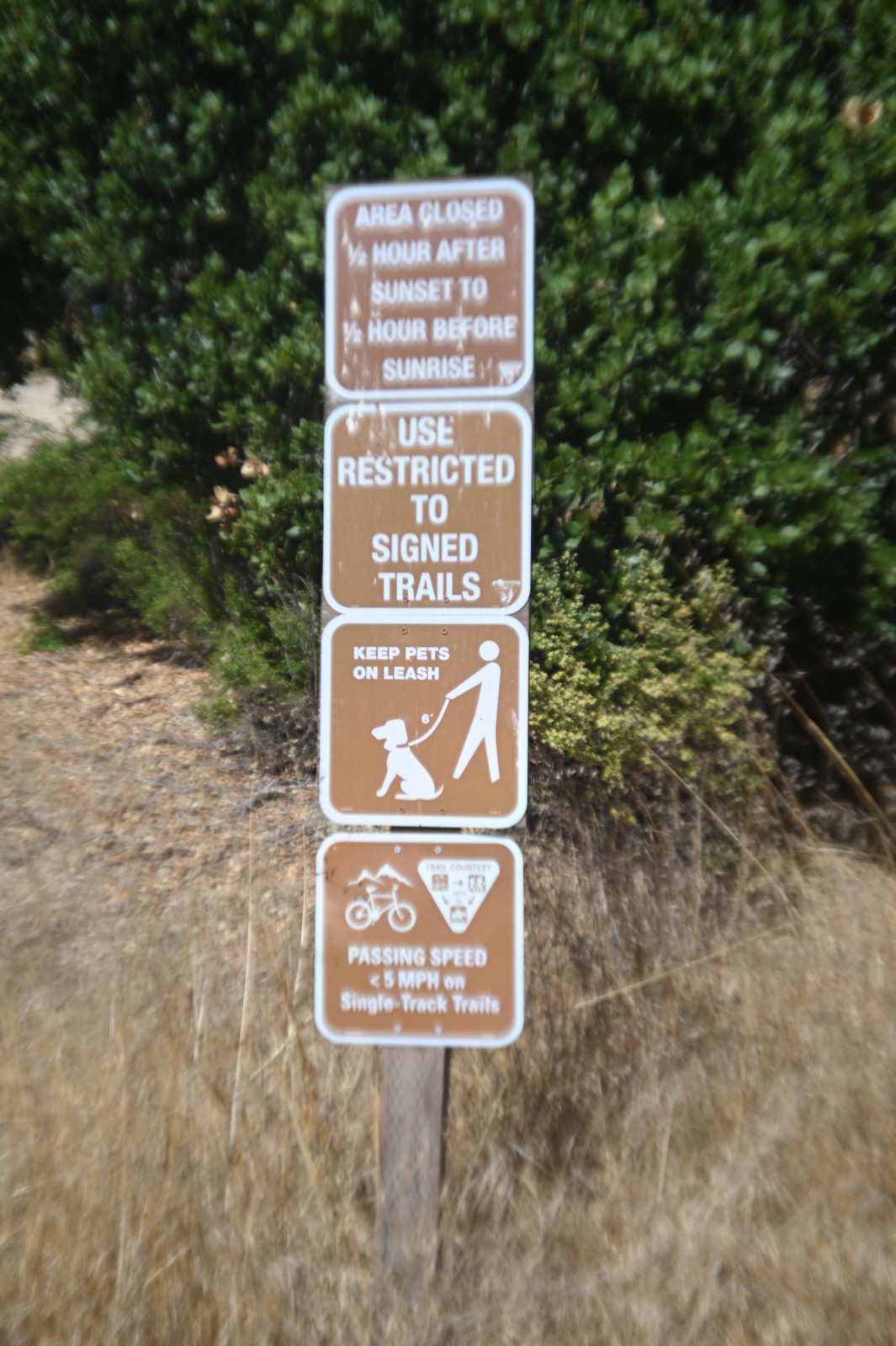This photo captures a weathered wooden post rooted in a patch of dry, brown grass, and it supports four small, square, brown metal signs outlined in white. Nestled in an outdoor setting under bright sunlight, there are lush green shrubs—one with yellow flowers—and some trees in the background. The first sign reads "Area closed half an hour after sunset to half an hour before sunrise." The second sign dictates, "Use restricted to signed trails." The third sign, featuring an illustration of a person walking a dog, states, "Keep pets on a leash." The final sign advises a "Passing speed of five miles per hour on single track trails" and includes an image of a bicycle and an upside-down triangle.